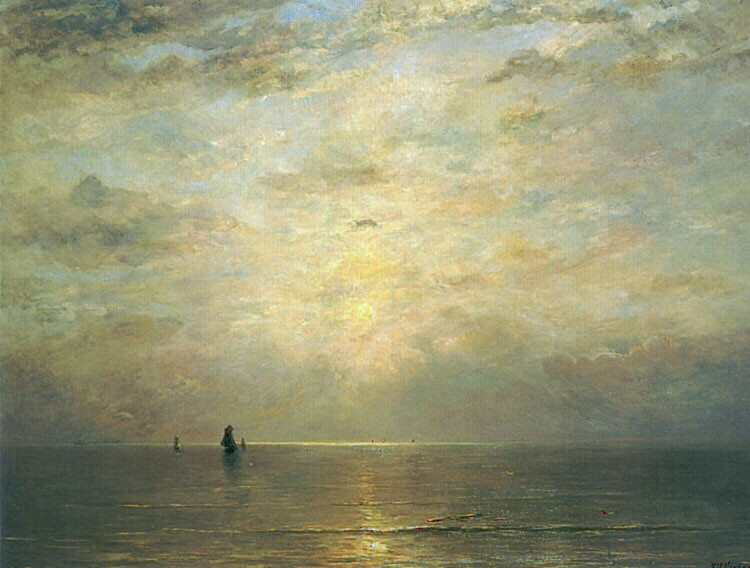The image is a painting, portraying an evocative seascape set during either sunrise or sunset, characterized by soft, diffused light. The bottom third of the composition is dominated by a grayish ocean, with gentle waves reflecting the weak sunlight that barely penetrates the cloud cover. In the distance, on the left side, three faintly discernible sailing ships—one larger than the others—are seen dotting the horizon. The middle of the painting features a faint sun obscured by clouds, casting a reflective path across the water, which stretches all the way to the viewer's perspective. The upper two-thirds of the image are filled with a dynamic sky, showcasing a mix of light blue hues, gray, and white clouds. The sunlight behind the clouds creates an ethereal effect, almost as if the light were spilling over the horizon line. Although there is a hint of an artist's signature in the lower right corner, it remains partially cropped and indistinct.